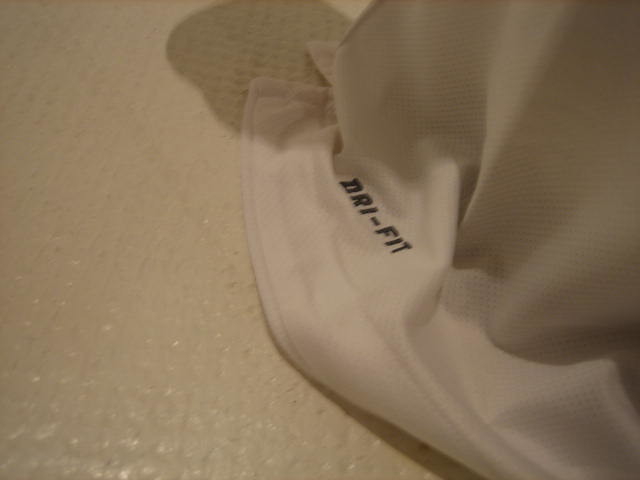The photo captures the edge of a white Dri-Fit t-shirt, prominently displaying the "DRI-FIT" label in black text. The t-shirt appears to be made of a soft, breathable athletic material with a grid-like pattern of stitches, indicating its high-quality construction. It is placed or possibly lying on a white, textured floor resembling a golf ball surface, characterized by small divots. The garment is folded with numerous wrinkles, and its careful craftsmanship is evident in the detailed threading. A distinct shadow stretches from the top right of the t-shirt towards the center of the photo, adding depth to the image. At the top middle section of the photo, a small slit is visible along the bottom side of the shirt, further showcasing its design elements.